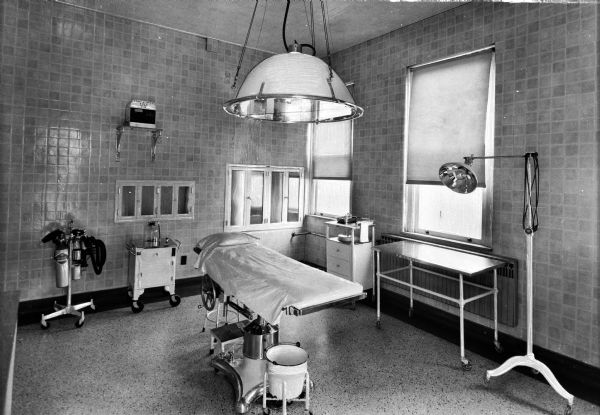This black and white photograph captures a vintage operating room, possibly from the 1950s, arranged in a landscape layout. At the center of the room, there is an operating table covered with a sheet and a pillow, accompanied by a white trash can at its foot. Surrounding the table, various pieces of medical equipment and furniture are visible. In the right corner stands a light fixture, while nearby, a metal device on wheels equipped with oxygen tanks and a small table, possibly holding a glass, can be seen. Against one wall, there's a window with a shade partially drawn, allowing light to filter into the room, and below the window sits a table with white legs. A white cabinet is positioned next to the table. The room is characterized by its retro design, with speckled flooring and tiled walls, enhancing the nostalgic ambiance of this well-preserved hospital setting.